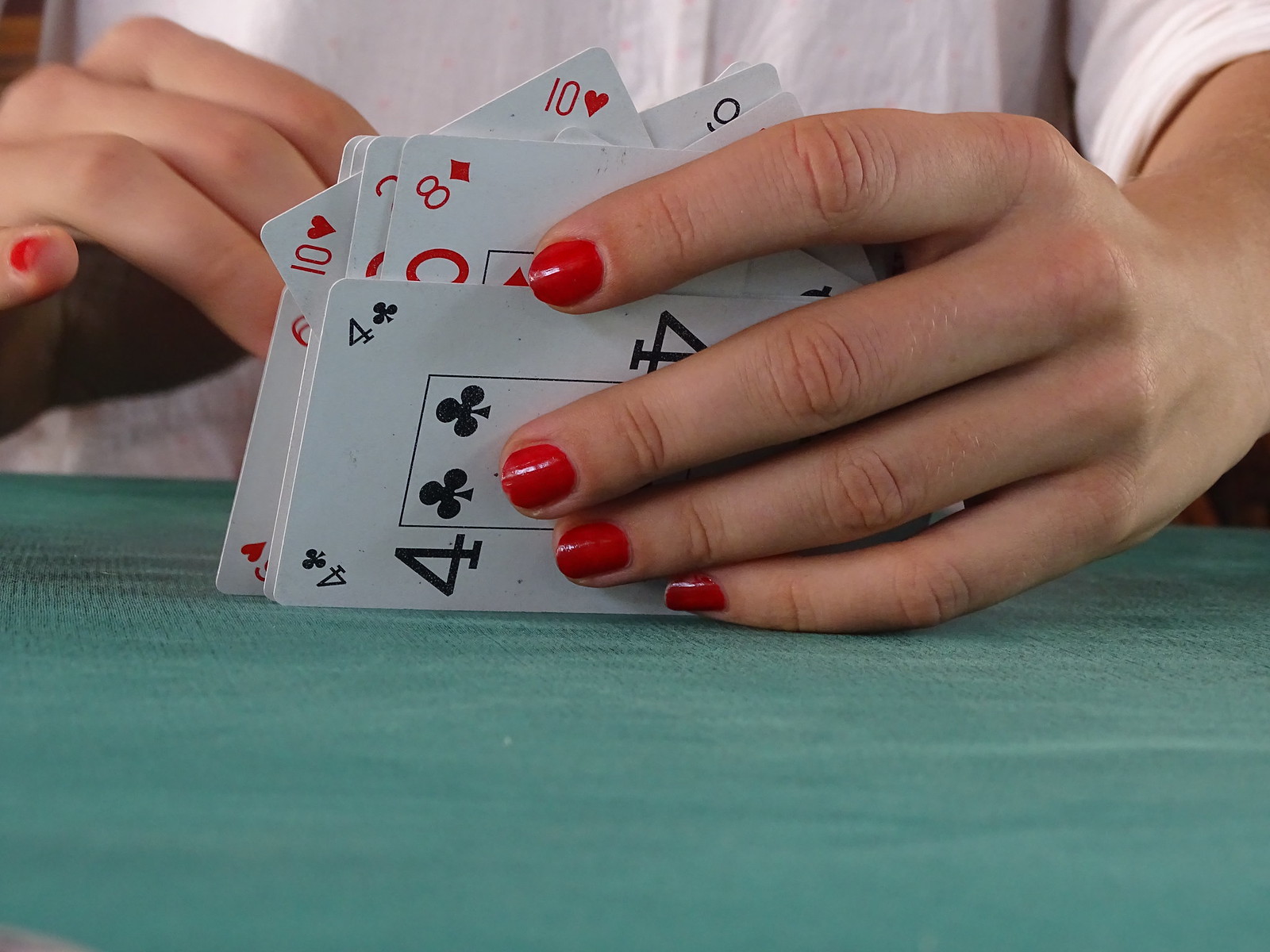A young woman, with vibrant red nail polish, is captured holding playing cards at a poker-style table draped in rich green velvet. She’s seated comfortably, wearing a plain white t-shirt that contrasts subtly with the vibrant table cloth. Her left hand holds a spread of cards, resting gently on the table while allowing a clear view of the card faces. Visible in her hand are the four of clubs, eight of diamonds, ten of hearts, and a few others. The playing cards themselves are of an unusual design with some numbers positioned diagonally, and the clubs, in particular, placed within a central box on the card. She appears to be in the midst of shuffling, and her hands suggest she is quite young.